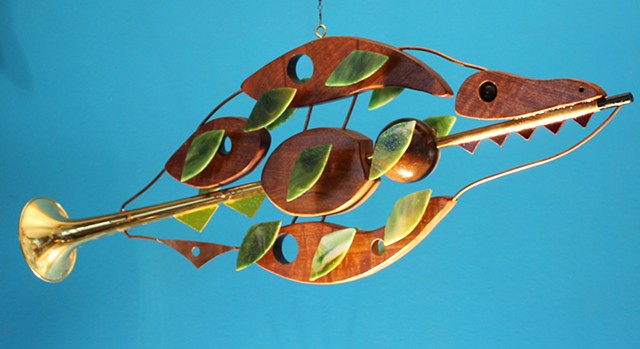The image features a meticulously crafted hanging wind ornament fashioned from a variety of materials, most prominently a modified gold-colored bugle. This artwork, which resembles a fish or perhaps a reptile, is foregrounded against a turquoise background. The side view reveals an elongated horn extending from right to left, with the flared end of the instrument on the left and the black mouthpiece nearly off the right edge of the image. 

Enhancing its fish-like appearance, the ornament includes intricate details such as a piece of wood forming the head, complete with a prominent black eye and nose. Below the head, five small, jagged pieces of wood mimic the appearance of sharp teeth. Along its body, thin copper wires frame the structure, and attached to these are several wooden pieces including one round and one oblong, adorned with green leaves that function as fins. The wood elements and green leaves provide a natural aesthetic against the metallic elements of the bugle and copper wire. 

Overall, the piece seems to be a creative fusion of musical instrument and organic forms, suspended as if hanging from the ceiling or mounted next to a wall, making for a visually striking and imaginative artwork.